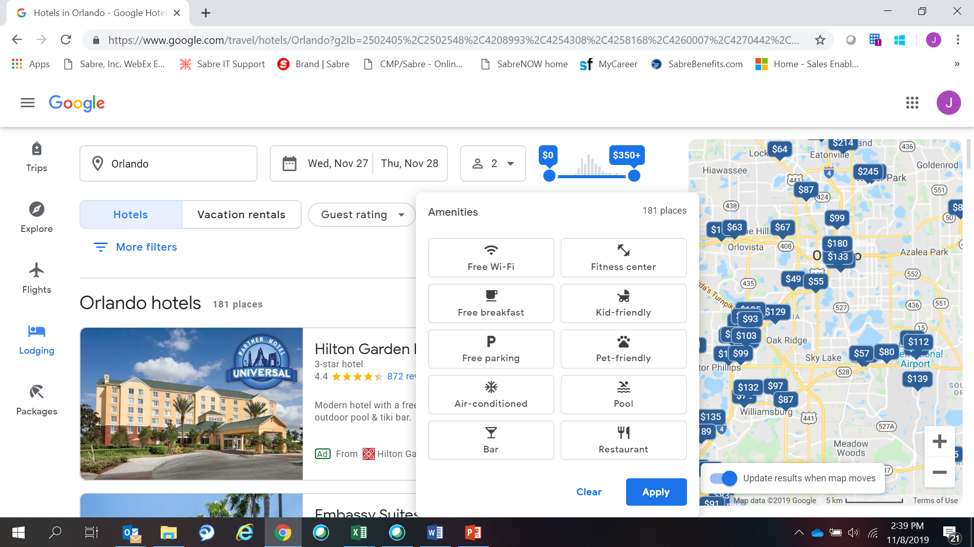The image depicts a Google Chrome browser displaying a Google search results page. The active tab is titled "Hotels in Orlando" and the browser's bookmarks bar is visible, containing several bookmarks labeled Sabre Incorporated, Sabre IT Support, Brand Sabre, MyCareer, SabreBenefit.com, and Microsoft Home. The search query appears to be focused on hotel accommodations in Orlando for the dates Wednesday, November 27th through Thursday, November 28th, for two people.

The search results prominently feature hotel options such as Hilton Garden, Orlando Hotel, and Embassy Suites. On the left side of the page, a menu is visible, listing categories like Trips, Explore, Flights, Lodging, and Packages from top to bottom. To the right, there is an embedded map displaying the Orlando area with various streets, ponds, and water sources clearly marked. Overlaying this map are numerous blue boxes indicating the locations and prices of hotels, ranging from $87 to $132.